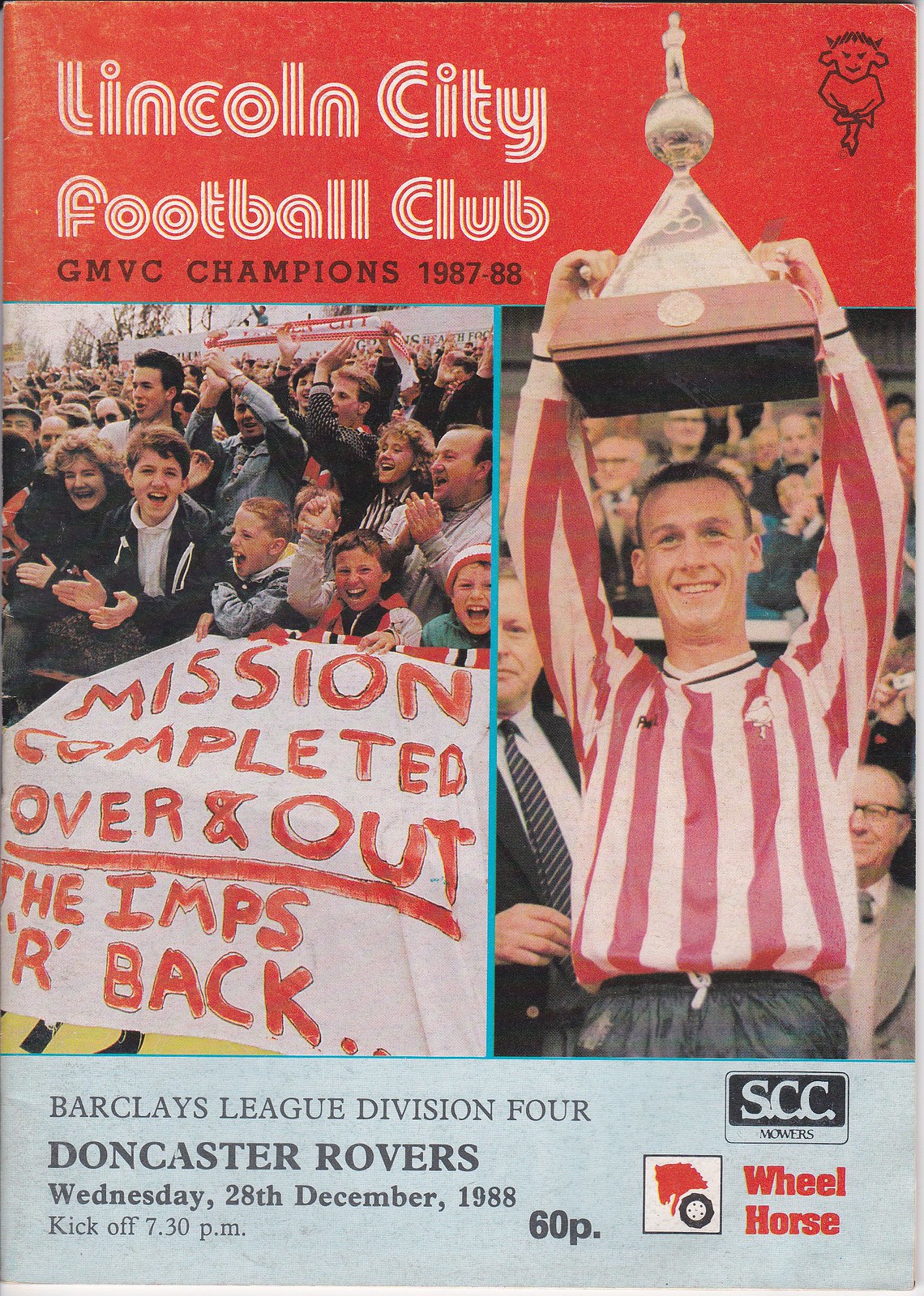The cover of the program booklet for the Lincoln City Football Club features a vibrant red background, with two main photographs capturing the celebratory atmosphere. On the left, a crowd of enthusiastic fans, including many children and adults, are cheering, clapping, and smiling. They are holding a large banner that reads, "Mission Completed, Over and Out, The Imps Are Back." On the right, a player in a red and white striped long-sleeve shirt is triumphantly holding up a large pyramid-shaped trophy adorned with a soccer ball and a figure on top. The top text of the cover proudly states, "Lincoln City Football Club GMVC Champions 1987-88." At the bottom, a gray horizontal stripe displays the match details: "Barclays League Division 4, Doncaster Rovers, Wednesday 28th December 1988, kickoff 7.30 p.m., 60 pence." Accompanying the text are logos for three sponsors: SCC Mowers, Wheelhorse, and a third logo resembling a soccer ball.